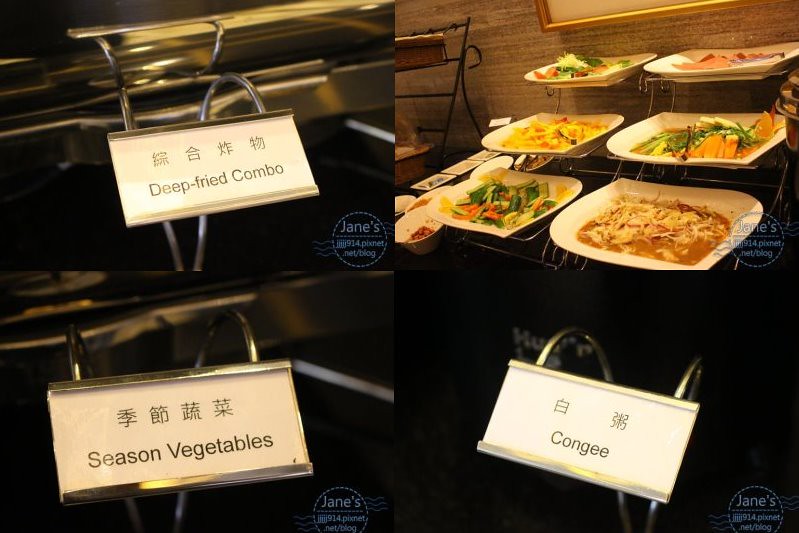This image is a detailed collage from a Chinese restaurant buffet, showcasing two distinct scenes side by side. On the left side, there are two place cards, one above the other, identifying the dishes as "Deep-Fried Combo" and "Seasoned Vegetables," with Chinese characters above each English label. These place cards are positioned in front of silver chafing dishes designed to keep the food warm. An additional detail at the bottom right of this side hints at the image source, marked as "James JJJ914.pixnet.net/blog."

On the right side, the focus shifts to a three-tiered shelving system displaying six different plates in total. Each shelf holds a variety of Chinese dishes, presented on a black table with a brown wall in the background. A prominent white plaque tags this section with the label "Congee" alongside corresponding Chinese text.